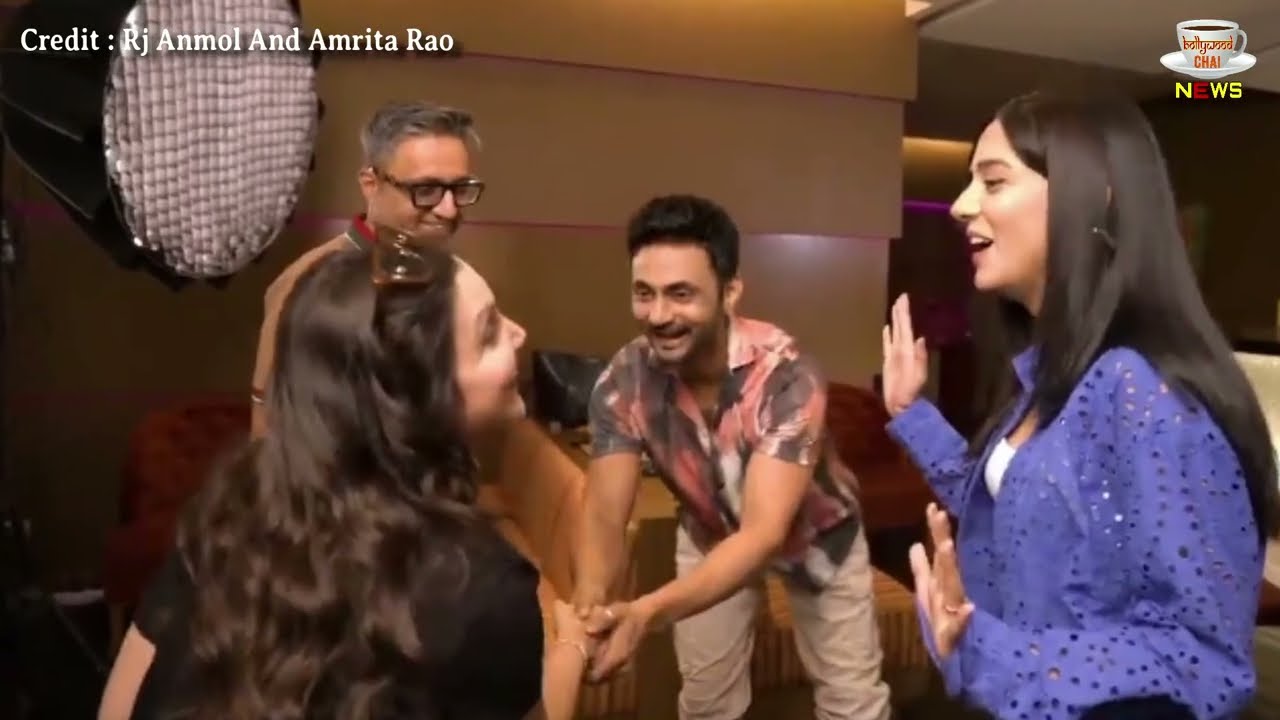An indoor image features a group of four people, seemingly of South Asian descent, laughing, smiling, and engaged in conversation. They stand before a brown-paneled wall, under a white object hanging from the ceiling on the left. The group consists of two women and two men. The woman on the far left has long, wavy dark brown hair, wears a black short-sleeve top, and appears animated, holding her hands up. Next to her, a man with short gray hair wears glasses and a brown sweater. The man next to him sports dark hair and wears a short-sleeve, button-down shirt in pink and gray hues with light khaki pants. The woman on the far right has long, straight dark brown hair, a purple sequined long-sleeve shirt with a white blouse underneath. In the upper left corner, a white font credit reads "RJ Anmol and Amrita Rao." A logo in the upper right corner comprises a white coffee mug and saucer with the text "Bollywood Chai" in a distinctive font, and below, the word "NEWS" in yellow letters except the 'E' which is in red.